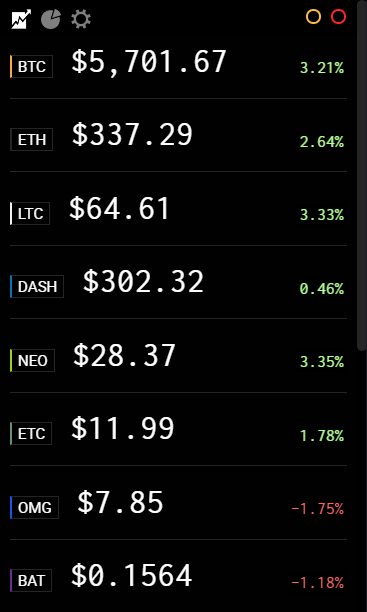The image in question is a detailed screenshot displaying Bitcoin and various cryptocurrency prices on a black background, formatted in a portrait, rectangular shape resembling a cell phone screen. There is no visible border surrounding the image.

In the upper left corner of the image, there are three icons: 
1. A white icon resembling a jagged upward-moving stock line inside a rectangular frame with a white arrow extending beyond the frame.
2. A gray circular icon resembling a pie chart with a segment pulled out.
3. A standard settings gear icon.

On the upper right corner, there are two empty circles; the left one has a yellow outline, and the right one has a red outline, both filled with the black background.

Below these icons, the image features a list of eight different cryptocurrencies, each formatted with three or four-letter abbreviations, current prices, and percentage changes. Here's a detailed breakdown:

1. **BTC (Bitcoin):**
   - Left Indicator: Orange vertical line
   - Price: $5,701.67 
   - Change: +3.21% (in green)

2. **ETH (Ethereum):**
   - Left Indicator: None clearly visible (possibly very dark)
   - Price: $3,377.29 
   - Change: +2.64% (in green)

3. **LTC (Litecoin):**
   - Left Indicator: White vertical line
   - Price: $64.61 
   - Change: +3.33% (in green)

4. **DASH (Dash):**
   - Left Indicator: Blue vertical line
   - Price: $302.32 
   - Change: +0.46% (in green)

5. **NEO (NEO):**
   - Left Indicator: Light green vertical line (matching the percentage color)
   - Price: $28.37 
   - Change: +3.35% (in green)

6. **ETC (Ethereum Classic):**
   - Left Indicator: Gray vertical line
   - Price: $11.99 
   - Change: +1.78% (in green)

7. **OMG (OmiseGO):**
   - Left Indicator: Royal blue vertical line
   - Price: $7.85 
   - Change: -1.75% (in red)

8. **BAT (Basic Attention Token):**
   - Left Indicator: Lavender vertical line
   - Price: $0.1564 
   - Change: -1.18% (in red)

Each cryptocurrency is presented in a well-organized manner, with its abbreviated code on the left followed by a much larger price in white, and ending with the percentage change on the far right. The percentage changes are color-coded: green for positive changes and red for negative changes.